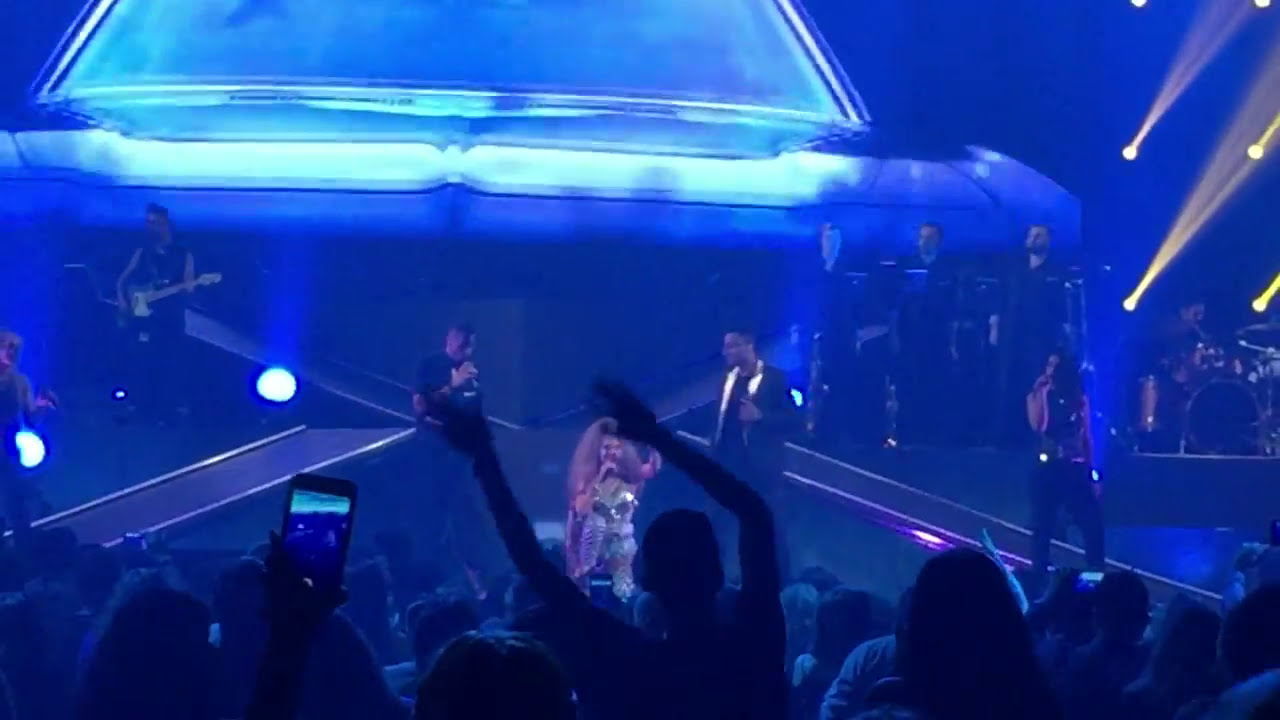The image depicts an indoor concert scene bathed in blue lighting, creating a surreal atmosphere. The stage is segmented into different levels, with the central focus being a woman in a silver outfit and big poofy hair, singing into a microphone while seated. Flanking her are two male backup singers, with additional musicians and singers positioned further back. To the left of the woman, a guitarist stands on the second level, and to the right, further back, there is a drummer illuminated by four upward-shining yellow beams of light. The backdrop features an image resembling the front end of a car, complete with a grille and windshield, giving it a UFO-like appearance. The audience in the foreground is shrouded in darkness, with only their outlines visible. Some members of the crowd are actively engaged, raising their hands, taking pictures and recording the performance with their phones. The entire scene is a dynamic blend of light, shadow, and music, capturing the energetic essence of a live performance.